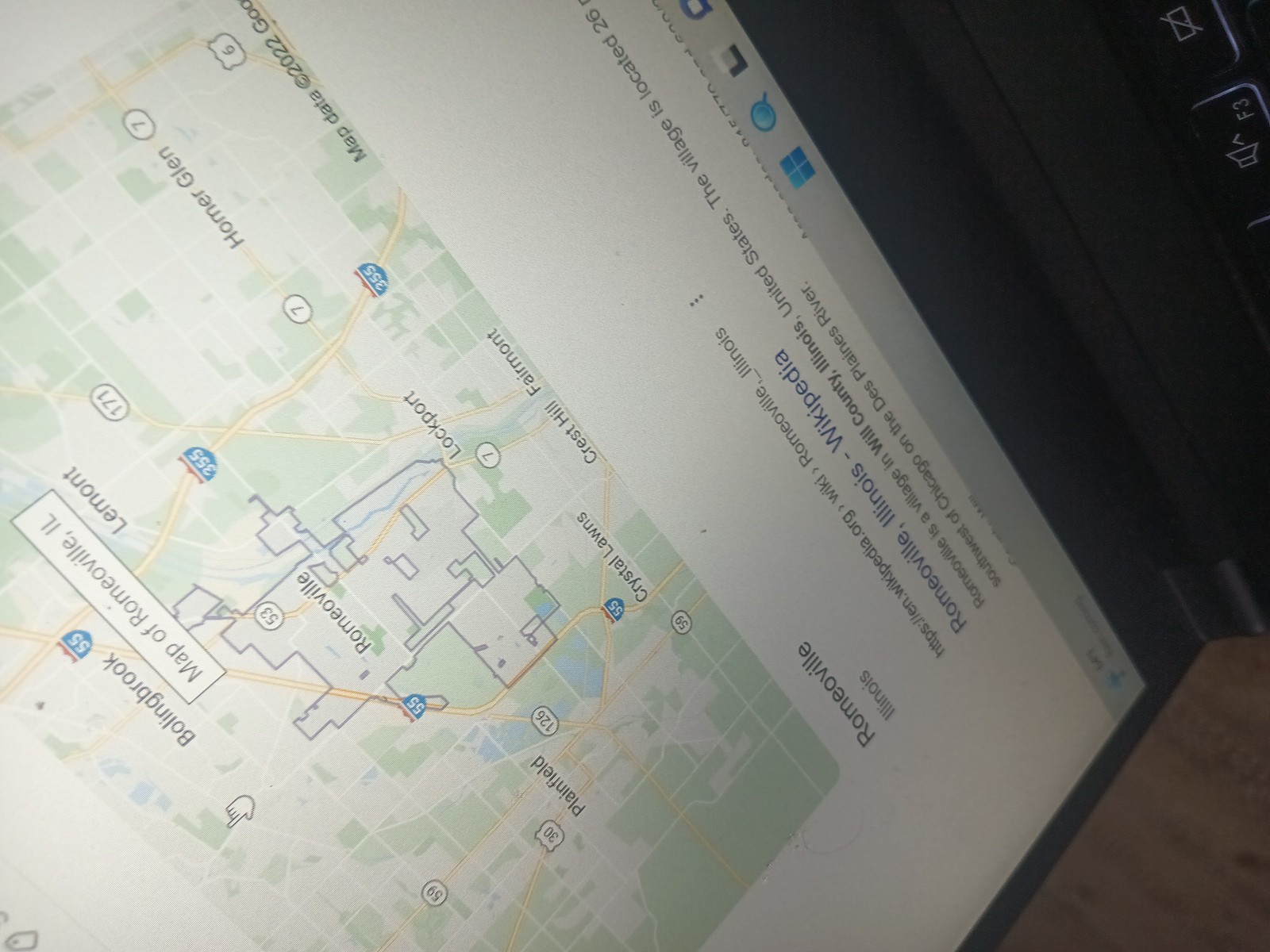This image appears to be a screenshot of a Wikipedia page or search results for Romeoville, Illinois. The page includes a detailed map of Romeoville from Google Maps, highlighting key routes such as Interstate 55, Route 53, and Route 7, which all intersect within the village. Romeoville is shown in proximity to several neighboring areas, including Plainfield, Crystal Lawns, Lockport, Lemont, Bolingbrook, Crest Hill, and Fairmount. The visible text on the page mentions that Romeoville is a village in Will County, Illinois, United States, and is located southwest of Chicago along the Des Plaines River.